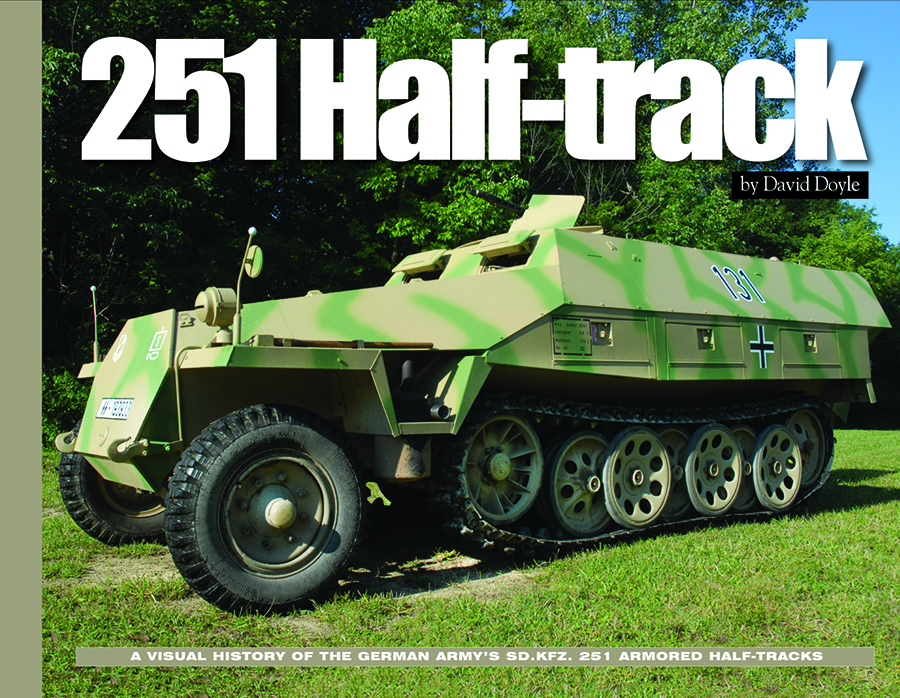The image depicts a military vehicle, specifically labeled as "251 Half Track" in large white letters at the top. Below this, it details "A Visual History of the German Army's SDKFZ 251 Armored Half Tracks" in white text on a black background. The author of this visual account is noted as David Doyle. This half-track vehicle is a blend between a truck and a tank, characterized by its distinctive structure: the front features two large truck wheels, while the rear is equipped with continuous treads, typical of a tank, to enhance mobility.

The vehicle's exterior is painted in a camouflage pattern with light and darker green streaks, suitable for forest environments. The body is fully armored with small, rectangular slits likely intended for defensive firing. The number "131" and a black cross with a white outline, a symbol of the German army, are printed on its side. This half-track is captured in a grassy field with large trees in the background, suggesting a daytime setting outdoors.